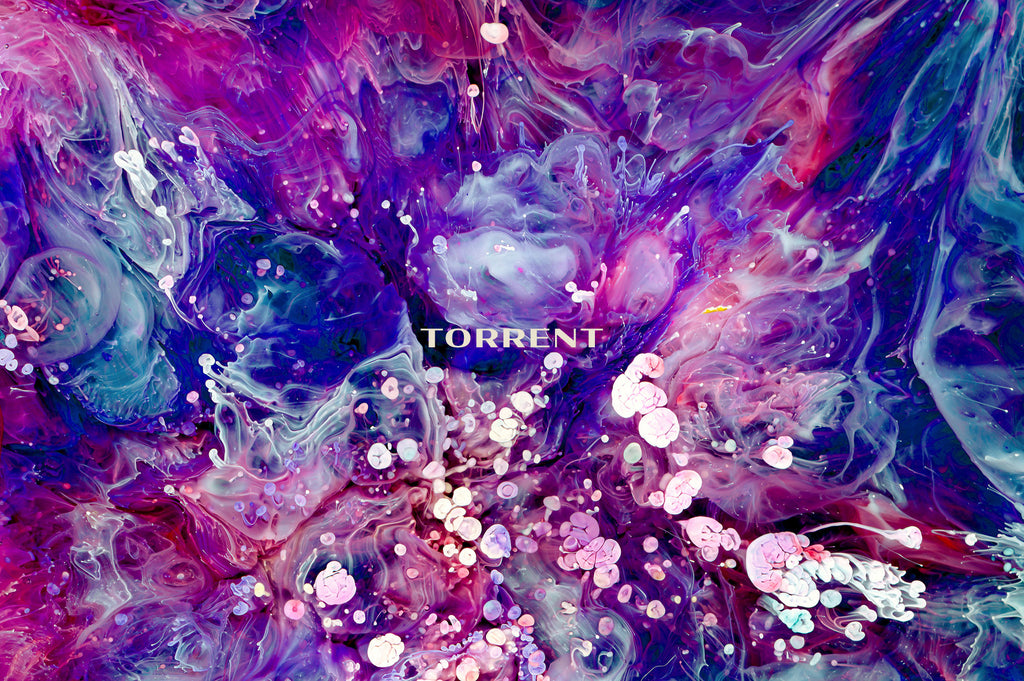The image is a vibrant and captivating advertisement for a brand named Torrent. Dominating the center of the image, the brand name "TORRENT" is displayed in white capital letters in a block typeset. The background is an intricate and artistic mix of swirling and splattering paint, giving a marbled effect. The color palette includes shades of dark pink, light pink, dark blue, light blue, along with purples, turquoise, and hints of yellow. The swirls and drips create a dynamic, ocean-like scene with some lighter circular areas that evoke images of coral or even the textures of a brain. The design stretches across a longer-than-tall canvas, making for a stunning and abstract screensaver or wallpaper. The overall impression is of a high-class, stylish brand, using a dazzling array of colors and fluid patterns to catch the eye.